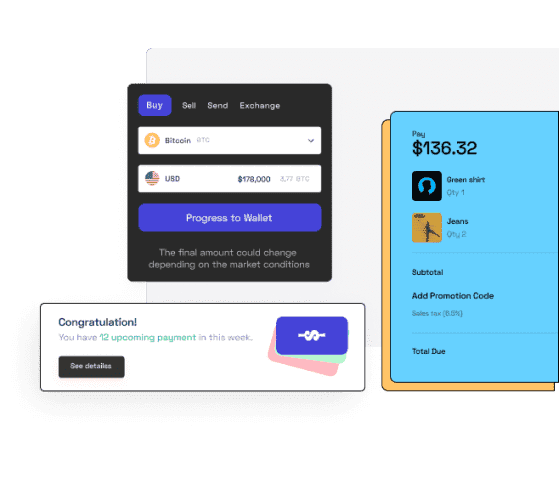In this image, we observe a detailed financial dashboard showcasing various cryptocurrency transactions and market activities. It prominently features options for buying, selling, sending, and exchanging Bitcoin (BTC) and USD, with a highlighted amount of $178,000 moving towards a recipient's wallet. Please note that this final amount is subject to change with market fluctuations. The user is notified of 12 upcoming payments scheduled for the week, with the option to view further details. On the right side, there's a breakdown of a payment for a green shirt, priced at $136.32, with a quantity of 1 for James and a quantity of 2 for another unspecified item. The subtotal is calculated before adding a 6.5% sales tax, leading to the total amount due. The user interface features a vibrant color palette, including black, blue, orange, white, yellow, and pink. Thank you for watching.